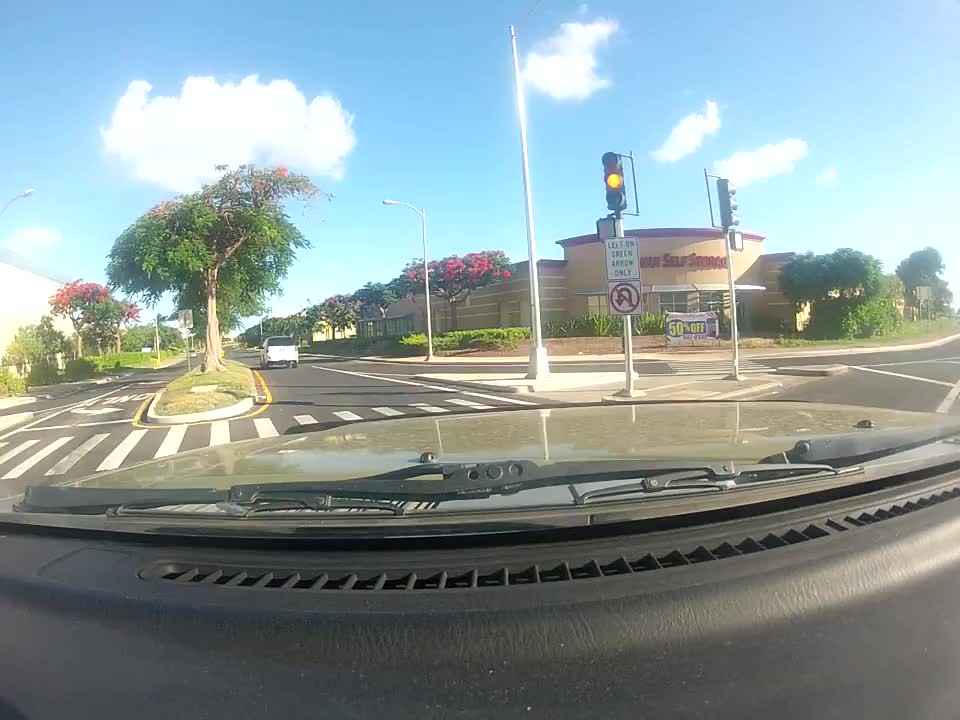This detailed image captures the view from inside a moving car, looking out through a clear windshield. The dashboard, with its gray surface and windshield wipers, is visible at the bottom. The focal point is the bright yellow traffic light suspended on a black steel post over the road, signaling caution. Just below this traffic light is a white sign, followed by a 'No U-turn' sign. To the left, a median of trees with some flowering varieties and green bushes separates the lanes, with sparse clouds dotting the vibrant blue sky above. The road beneath is gray asphalt, marked with white lines to indicate a crossing area. Off to the right stands a light brown brick building with red lettering on the front, possibly a store advertising a '50% off' sale. In the background, a white truck can be seen driving past this shopping center. Overall, the image captures a bright, sunny day with clear visibility and no pedestrians in sight.